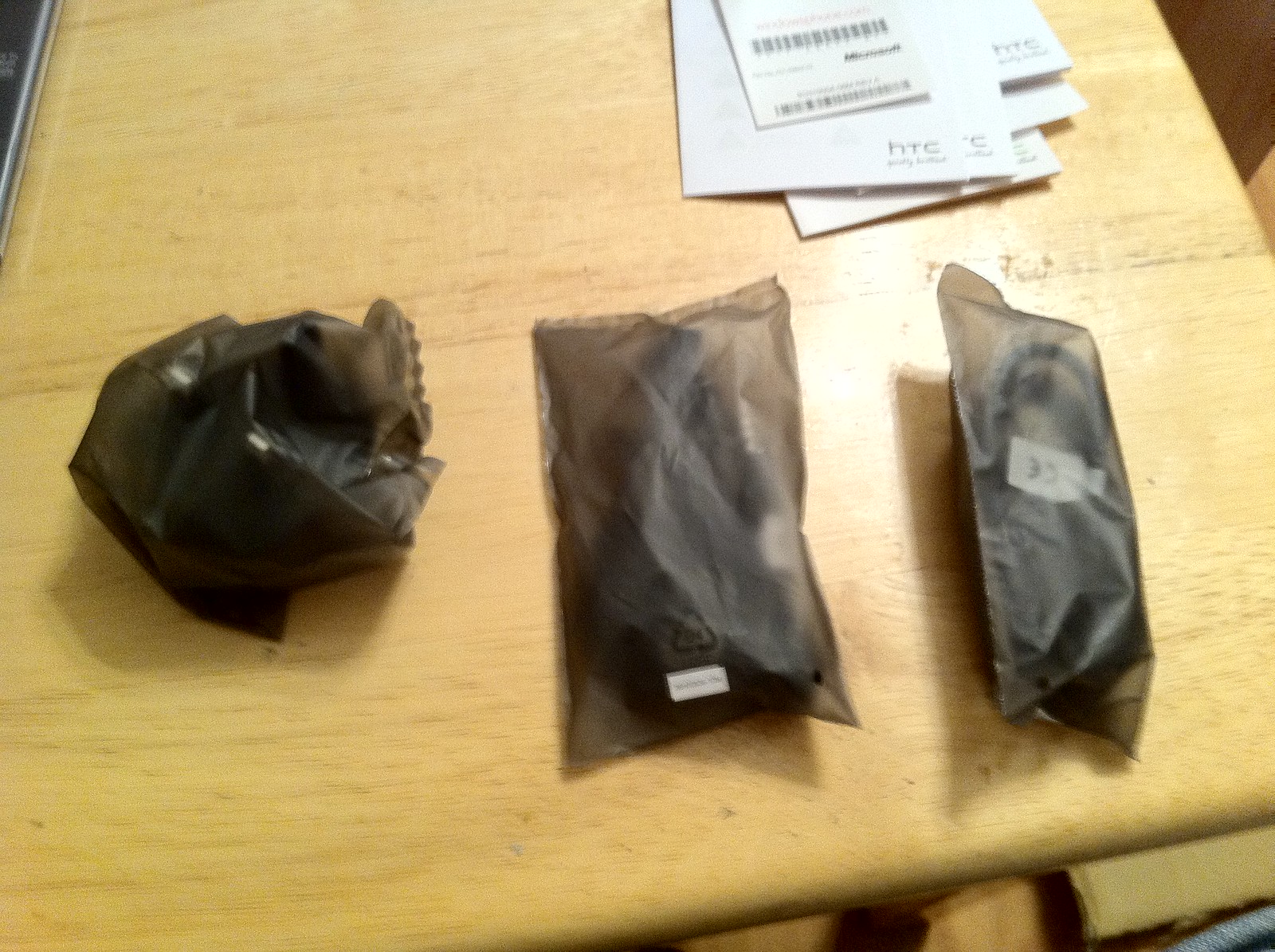In the photograph, there is a light brown, beach-colored wooden table that serves as the backdrop for the scene. The table hosts three black, slightly see-through plastic bags positioned closely together. The bag on the left is noticeably scrunched up into a ball, suggesting that its contents might be broken or malleable. The middle bag, displaying some wrinkles and a small white label at the bottom, stands upright and is less distorted. The right bag is tilted slightly away from the viewer, revealing a visible cable inside. Besides the bags, there is a stack of papers or manuals on the table. Among these, a manual prominently displays the word "Microsoft" along with a barcode and some text, while another manual is identifiable as an HTC manual. The image's overall quality is low, hinting it might have been taken with a lower-end device.